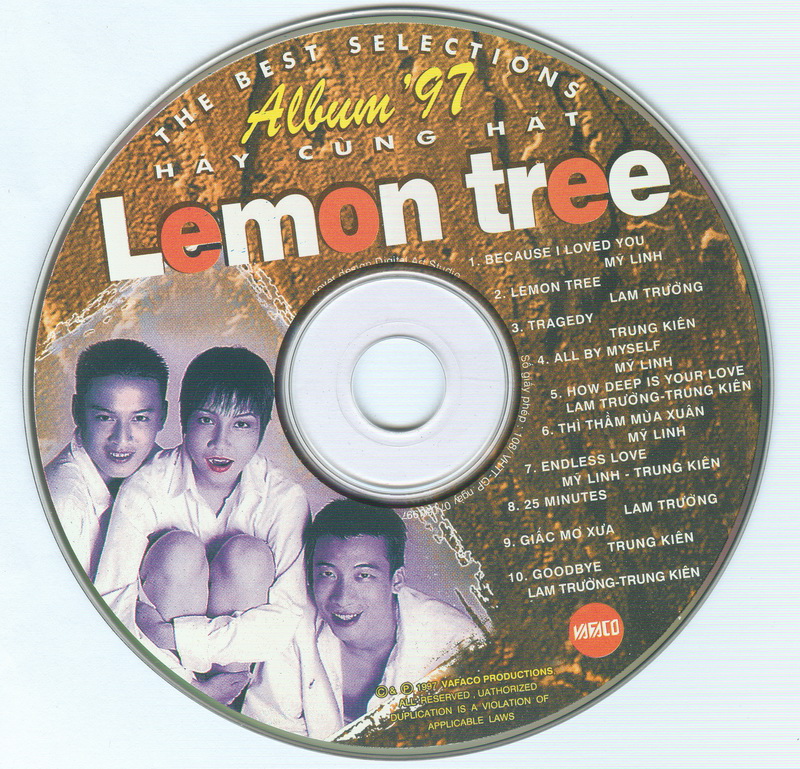The image captures a detailed close-up of a CD against a light blue background. The CD itself has a brownish backdrop with intricate text and visuals. At the top, in white letters, it reads "The Best Selections," followed by "Album 97" in bold yellow letters. Below it, in a mix of white and red letters, is the title "Lemon Tree," with the letters 'E' and 'O' in red and the rest in white. On the right-hand side, a list of ten song titles appears in white letters, starting with "Because I Loved You" by Mai Lin and including other tracks like "Lemon Tree" by Lam Truong, "All By Myself" by Mai Lin, and "How Deep Is Your Love" by Lam Truong and Trung Kien, among others. 

The left side of the CD features an image of three people, two men and one woman, all dressed in white dress shirts with dark hair. The woman, positioned in the middle, is notable for her red lipstick and appears to have fang-like vampire teeth. The entire trio is enclosed within a slightly worn, purplish box. At the bottom right corner of the CD, there is a red circle with "Vafeco" in white letters, indicating the production company. Additionally, copyright information in yellow letters surrounds the CD, stating "1997 Vafeco Productions. All rights reserved. Unauthorized duplication is a violation of applicable laws."